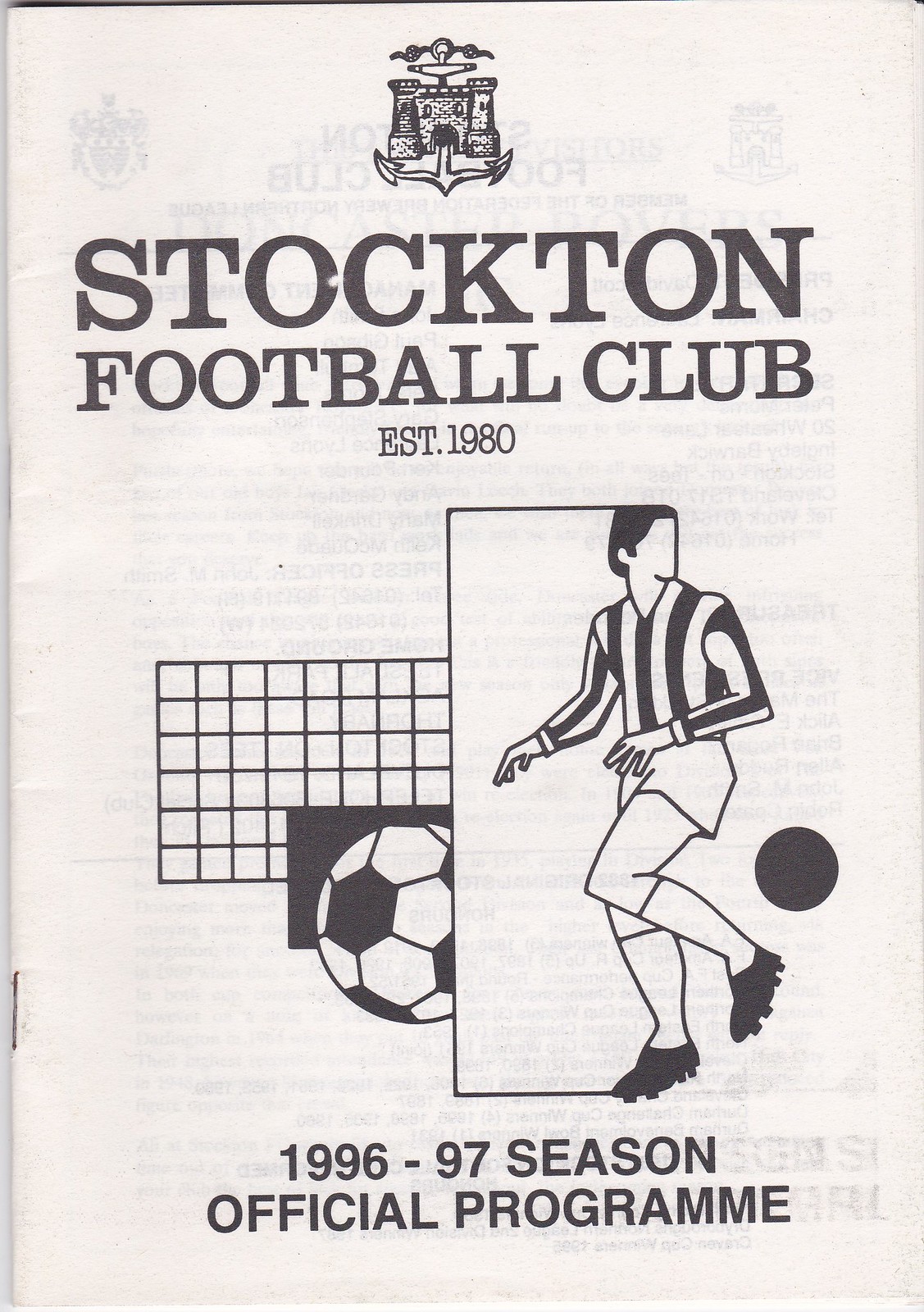The black and white cover of the Stockton Football Club's official program for the 1996-97 season prominently features detailed graphics and text. At the top of the cover, "Stockton Football Club Established 1980" is written, accompanied by a small logo of a castle. Below this, a line drawing depicts a soccer player dressed in a striped black and white long-sleeve jersey, white shorts, and black cleats, as he kicks a black soccer ball. Adjacent to him are additional graphics of a soccer ball and a net symbolizing a goal. The caption at the bottom of the cover reads "1996-97 Season Official Program."